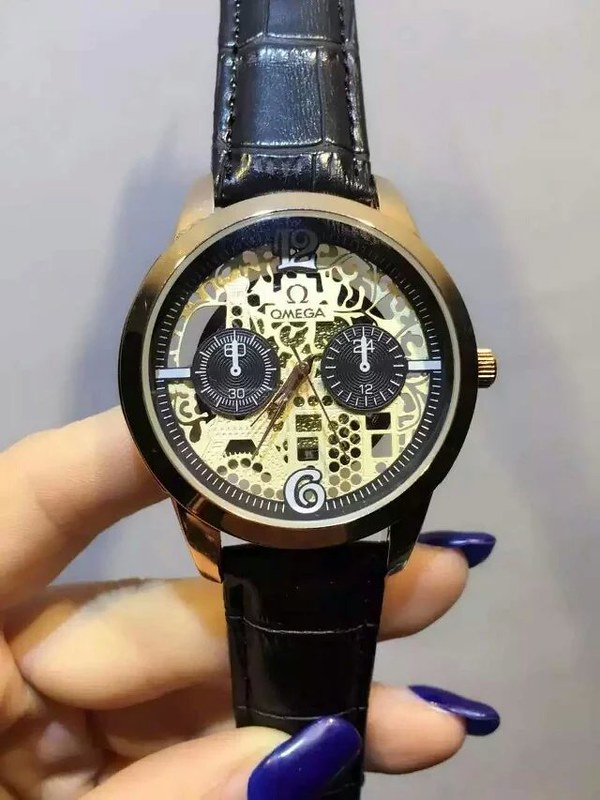This color photograph, likely taken under professional studio lighting, showcases a close-up view of a woman's left hand with manicured, royal blue nails, holding an intricate Omega watch. Her thumb is positioned across the black leather band, while her index finger is placed behind the gold-framed watch face, allowing the rest of the watch to drape over her remaining fingers. The sophisticated watch features a gold face with a stenciled background, through which some of the watch's inner mechanics are visible. Prominently displayed on the face are the Omega brand name and logo. The watch face exhibits large, whimsical numbers 12 and 6, while two smaller dials, flanked on either side of the watch center, indicate secondary functions; one dial shows the numbers 60 at the top and 30 at the bottom, and the other shows the numbers 24 above and 12 below. The background behind the hand and watch is white, and the watch's reflective surface creates a subtle reflection on the backdrop.